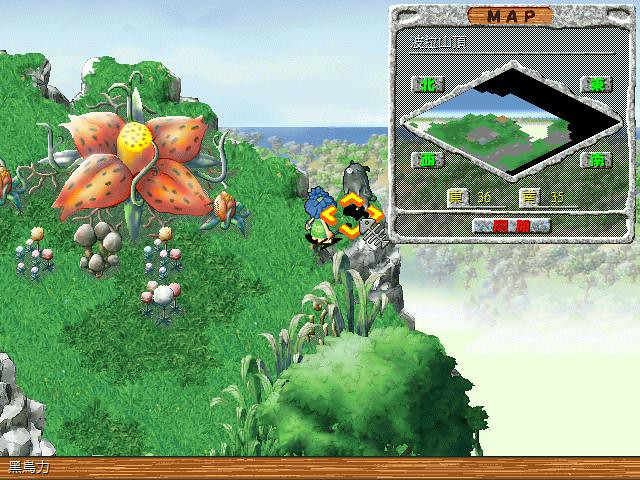This screenshot captures an isometric view of a classic Japanese RPG with pixelized graphics, reminiscent of retro console games from the early 90s. At the center of the scene stands a character outfitted like a caveman, sporting a primitive green outfit and distinctive blue hair, facing away from the camera. In front of the character is what appears to be either a statue of a pig or an actual pig, ambiguous in its stillness. 

To the left, a striking orange flower with black-spotted petals and a vivid yellow center dominates the grassy terrain, encircled by smaller mushrooms. The landscape reveals a dense jungle or wooded area, gradually descending towards a vast ocean visible in the far background. Additional scenic elements include trees and a subtle fog drifting to the right. 

In the top right corner of the screenshot, a mini-map aids navigation, displaying explored and unexplored areas, marked with icons and numbers such as “36” and “35.” An overlay of Japanese text further suggests the game’s origin. The overall composition, from the verdant cliffside to the expansive valley and ocean, enhances the immersive adventure feel of this retro video game.